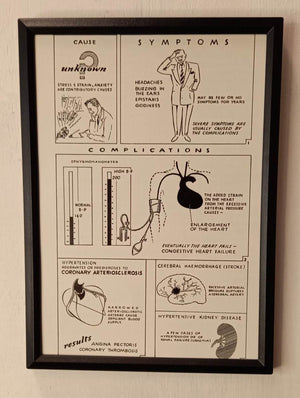This image is an old black-and-white framed medical diagram, likely from the 1960s, often found in a doctor's office. The frame is a basic black one, possibly from Walmart, and hangs on an off-white or eggshell-colored wall. The diagram itself, showing signs of age with a slightly faded white or beige hue, is divided into five distinct boxes filled with tiny, dense text. The first box, titled "Cause Unknown," features a small picture of a man with a large question mark, indicating an unknown cause for his condition. The second box, labeled "Symptoms," portrays a man in a suit holding his head, suggesting symptoms like a headache. The middle box, "Complications," depicts a person having their blood pressure taken, with an accentuated heart, implying elevated blood pressure affecting the heart. The bottom left quadrant mentions "Coronary Atherosclerosis," and there's an additional box showing a brain. This diagram presumably outlines the medical condition of high blood pressure and its impacts on various organs, such as the heart, brain, and possibly the kidneys, along with some suggested remedies and instructions for managing the condition.